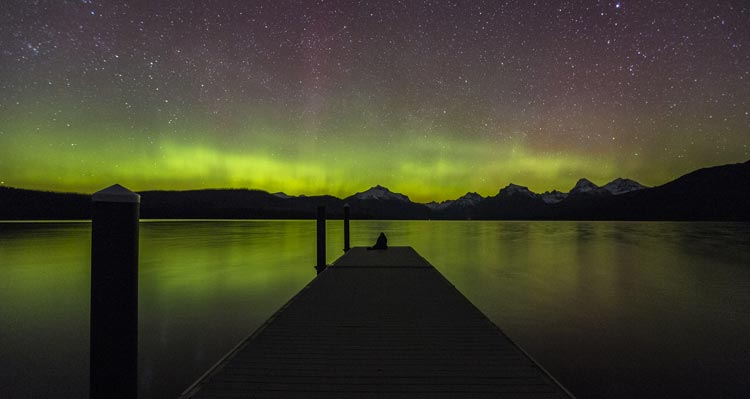The painting portrays a tranquil nighttime scene centered on a wooden dock that stretches from the lower center and lower right of the image towards the background, becoming smaller with perspective. The dock appears dark, almost silhouetted, under the night sky. A small, pointed-top tower and cylindrical posts line the left side, possibly for tying boats. The water in the foreground is a light brown, transitioning to a reflective lime green towards the center as it mirrors the greenish northern lights. Beyond the dock, a person sits at the end, grounding the scene in a moment of quiet contemplation as they gaze at the sky. The horizon features a horizontal range of mountain peaks bathed in a lime-colored glow, which contrasts with the dark, star-studded sky above. The entire image, rectangular and wider than it is tall, captures the serene interplay of natural elements under the mysterious night sky.